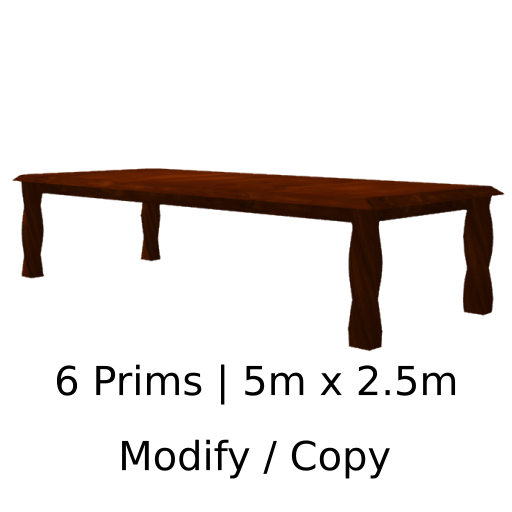The image features a detailed rendering of a long, low, rectangular coffee table. The table is a dark brown color, resembling mahogany, with a lighter brown tabletop. Its four legs, twisted and sculpted, widen and narrow before ending in square bases. The background is plain white, allowing the table to stand out clearly. Below the table, in bold black text, it reads "6 PRIMS | 5M X 2.5M". The term "prims" is unclear, but it quantifies the table in some way. Beneath this line, "MODIFY / COPY" is prominently displayed, indicating the table's status or attributes.